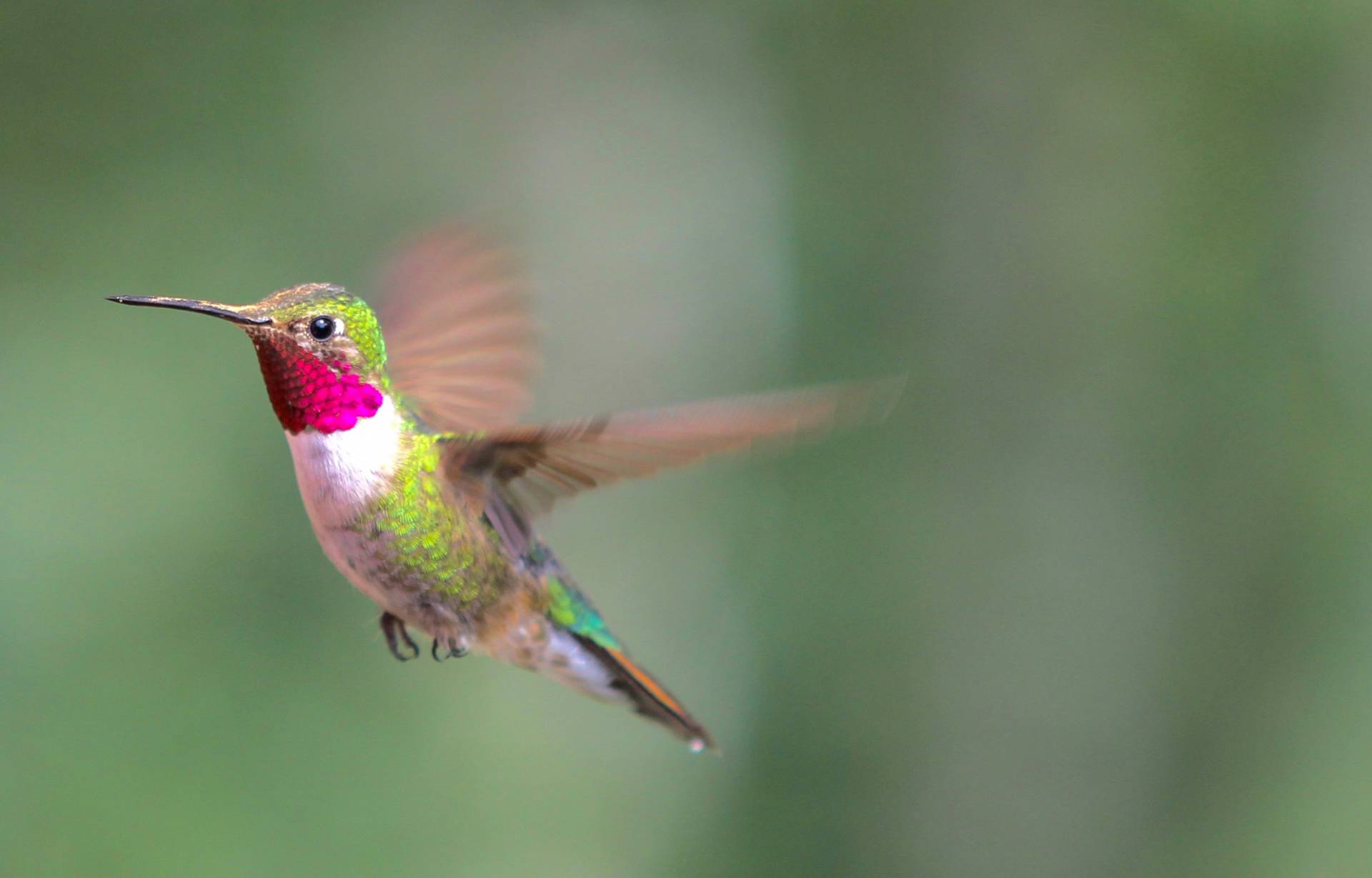The image depicts a stunning close-up of a hummingbird in mid-flight, captured with remarkable detail against a blurred background of greens and whites, likely foliage. The hummingbird occupies the left side of the frame, flying to the left, with its wings a blur from their rapid movement. Its long, pointed black beak is prominent, and its shiny black eyes add a hint of intensity to its focused expression. 

The bird's head transitions from grey at the top to a vivid fluorescent green streak over its eye, while its chin and cheeks display a bright red hue. Adjacent to its red chin, the lower neck is adorned with hot pink feathers, gradually blending into the white of its breast. This white coloration runs down to the base of its tail, which features a mix of black, orange, and a hint of bright blue tones. The side of its body glows with vibrant green feathers, adding to the overall iridescent appearance. 

The wings, barely discernable due to their speed, appear to have a reddish tint, merging with the dynamic energy of the scene. This picturesque moment, with its rich palette of pinks, greens, whites, and splashes of other colors, beautifully encapsulates the delicate beauty and agility of the hummingbird in its natural habitat.